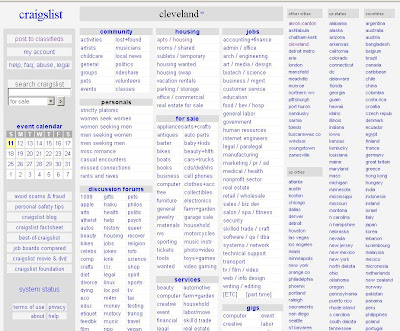The image primarily consists of a screenshot from a Craigslist webpage. 

In the upper left corner, the word "craigslist" is displayed in blue lowercase letters. To the right of this, there is a gray rectangle containing the city name "cleveland" in black lowercase letters. Below these elements, there is a series of categories listed vertically. These categories include: "community," "personals," "discussion forums," "housing," "for sale," "services," "jobs," and "gigs." 

To the right of these categories, there are four dark gray boxes, each containing some blue text beneath them, although the text is not legible. 

On the left side of the image, just under the "craigslist" logo, several links are displayed. These links include "post to classifieds," "my account," "FAQ," "abuse," and some other unreadable text. Below this, there is a search box labeled "search craigslist." 

Further down the left side, an "event calendar" is visible. Within this calendar, the date "Sunday the 11th" is highlighted in yellow.